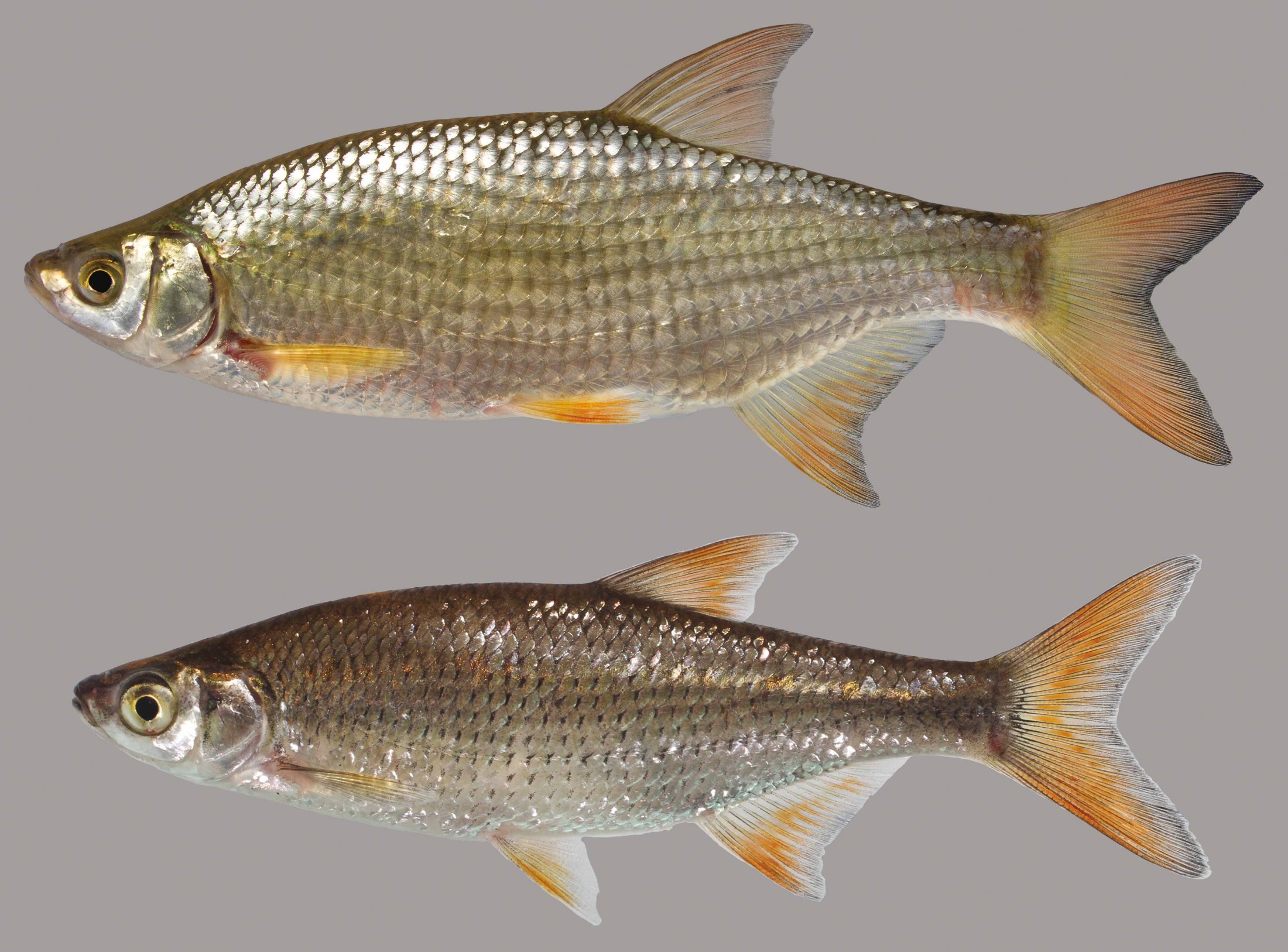This image features a close-up of two similar fish placed against a soft gray background. The fish appear to have been digitally cut out from another setting and placed onto this backdrop. Both fish are of the same species and exhibit primarily silver metallic scales that shimmer against the gray. Each fish has a distinct orange-red spot at the base of its gills and translucent fins tinged with yellow-orange hues, extending to their tail fins which also display hints of gray. The fish are oriented one above the other with a small gap in between. The top fish boasts golden scales interspersed with more silvery ones and seems to have a slightly greenish tint, while its dorsal area appears shadowed. The bottom fish is somewhat smaller and presents a darker, almost burnt orange coloration on its fins and tail. It is generally darker in shade, leaning towards a brown tone, and has a noticeably larger eye compared to the top fish.